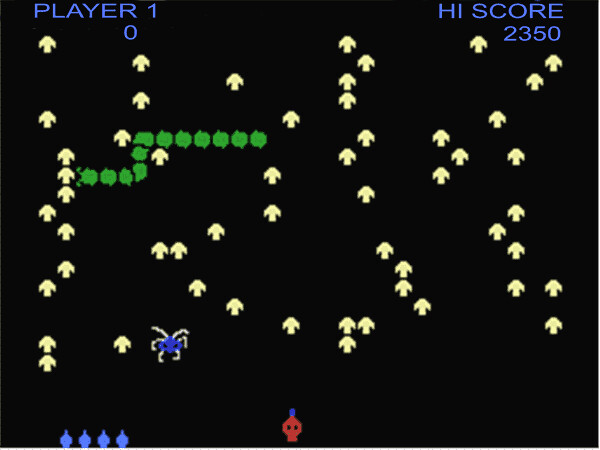This screenshot captures an intense moment from the classic arcade game, Centipede. The interface prominently displays "Player One" in blue letters at the top, with the current score set at zero and an all-time high score of 2350. In the game field, a vibrant green centipede, segmented into multiple pieces, winds its way through an intricate maze of small yellow arrows pointing upwards. A spider is descending from the top of the screen, adding to the challenge. Positioned at the bottom, the player's shooter is primed and ready to fire at both the centipede and the approaching spider. Additionally, four extra shooters are lined up at the bottom, indicating four remaining lives or turns. The screenshot vividly captures the game's dynamic and colorful graphics, as well as the strategic elements faced by the player.